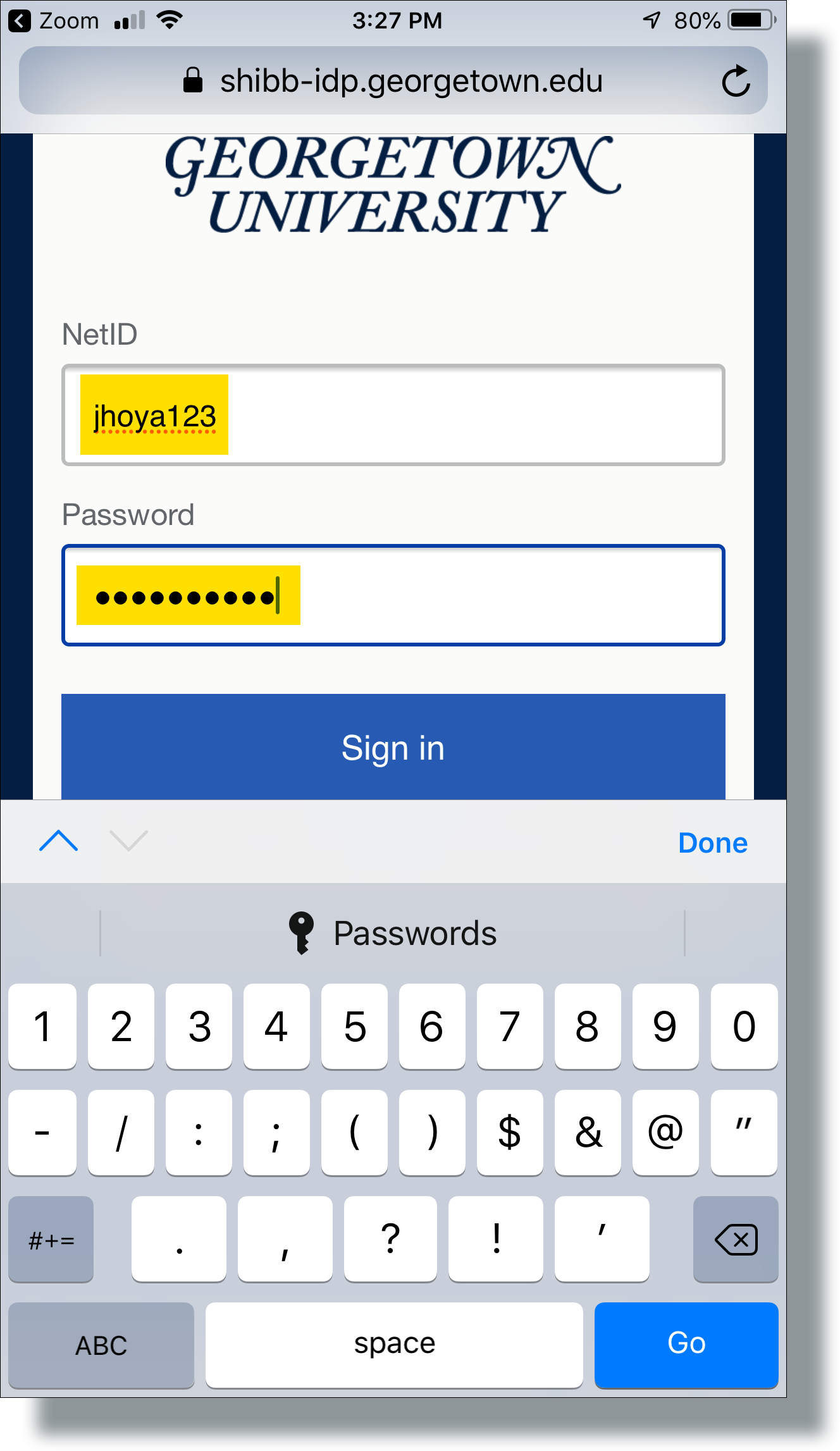A screenshot of a smartphone displaying an application interface. The status bar at the top shows the carrier signal strength at 2 bars, Wi-Fi is enabled, the current time is 3:27 PM, location services are active, and the battery level is at 80%. The Zoom application is also open in the background. A secure web address, indicated by a lock icon, reads "shib-idp.georgetown.edu" accompanied by a refresh arrow.

The screen prominently features the login page for Georgetown University. The header is in an elegant, descriptive blue font against a pristine white background. Below the header, a "NetID" input field is highlighted in yellow with bold black text displaying "JHOYA123". Adjacent to it is a long gray password input box, also highlighted in yellow, indicating that the password is being entered securely. At the bottom of the screen, the "Sign In" button is visible. Beneath the form, a virtual keyboard with numerical and alphabetical keys is present, facilitating user input.